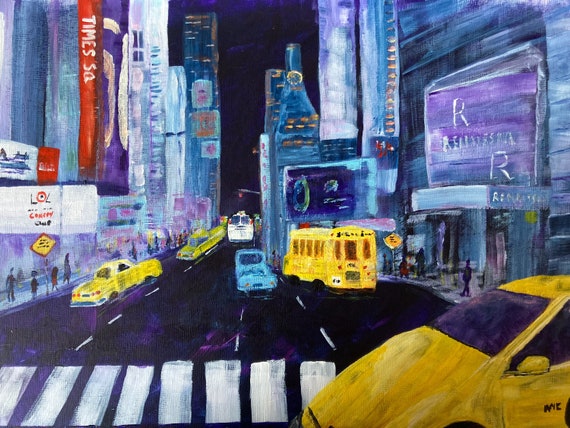This is a detailed painting of a nighttime street scene in New York City's Times Square. The composition prominently features three bright yellow taxi cabs and two buses – one resembling a school bus and the other a city bus. All are rendered with visible paint strokes, giving a rudimentary and dynamic feel to the scene. A large crosswalk marked by white vertical lines is situated in the foreground, while people are depicted standing or walking along the sides of the street.

The background is filled with many towering high-rise buildings and skyscrapers, all painted in various shades of blue, accented with a few red and white details. Large billboards and storefronts line the sides of the street, contributing to the bustling atmosphere of Times Square. Notably, a sign vertically reads "Times SQ" on one of the buildings on the left. On the right-hand side, a billboard featuring the letter "R" twice within a purplish-gray rectangle stands out. The overall color palette of the artwork is dominated by blues, adding to the nighttime ambiance of the scene. An awning or ceiling that juts out in the middle left reads "LOL something studio," reminiscent of a cinema sign.